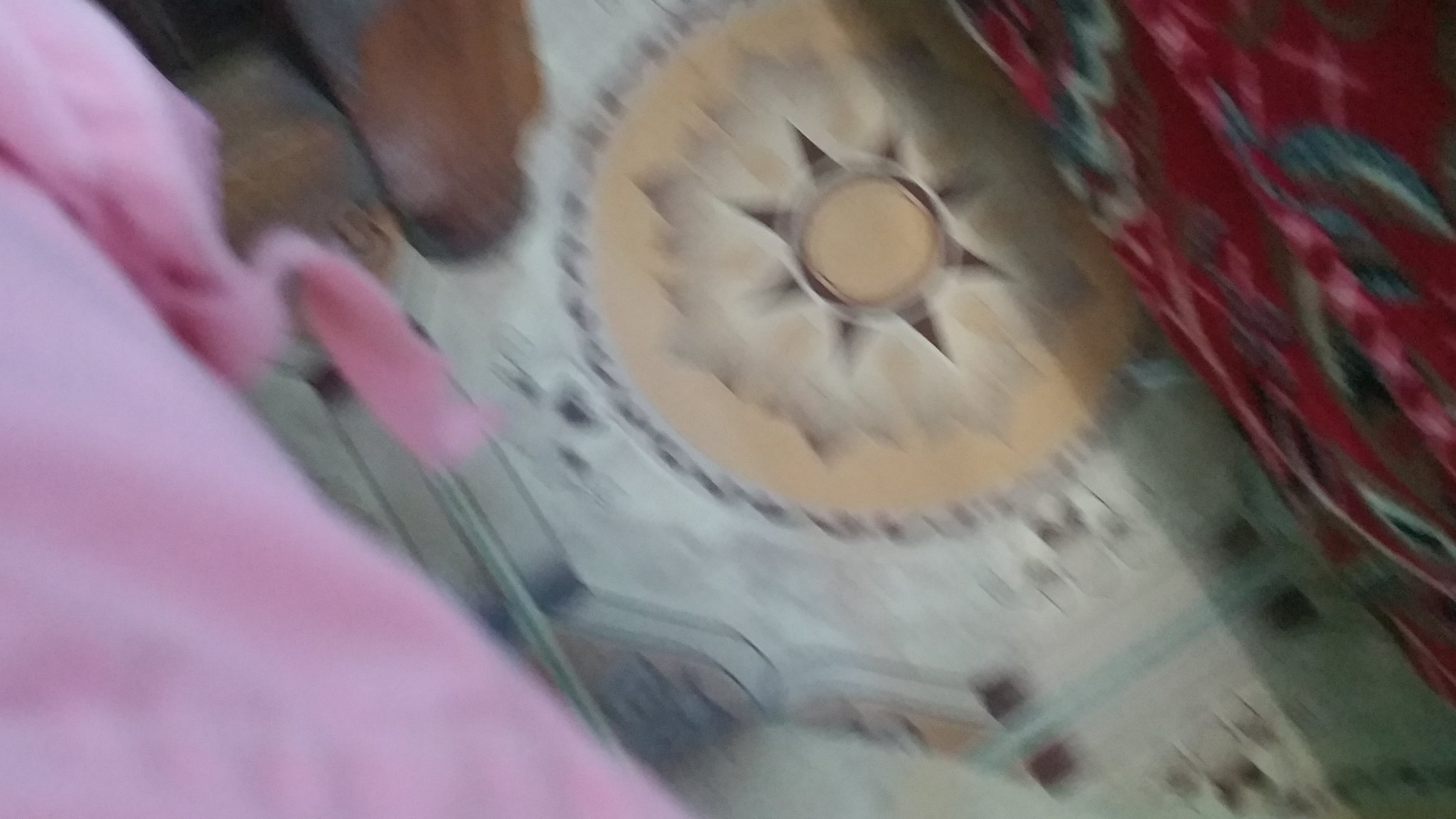The image displays a very blurry, motion-captured photograph that appears to be taken from above, possibly by accident. The scene seems to be inside a room, with the floor prominently featuring intricate tile or vinyl linoleum patterns. The most visible pattern is a detailed design resembling a brown sun with darker rays, surrounded by various circular borders.

To the left of the image, there is pink material that could be a person's leg or perhaps someone sitting on a chair. This pink fabric extends diagonally across the frame from the bottom center towards the top left. Nearby, there is a suggestion of wooden legs, likely from a piece of furniture, or possibly the closed tops of worn shoes.

On the right, a section of red floral-patterned fabric is visible, indicating part of a couch or another piece of fabric-covered furniture. This fabric section extends from the bottom right towards the center top, adding a potential Christmas-themed vibe with its brighter red tones and possible holly leaf patterns. The overall effect suggests a domestic scene with various elements captured in a state of motion, adding to the image's blurred and chaotic presentation.